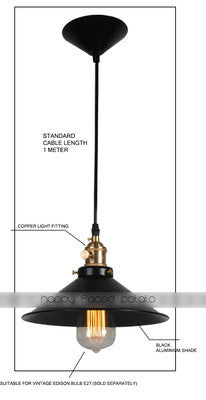This detailed illustration showcases a simple yet elegant hanging lamp designed with a standard cable length of one meter. The lamp features a copper light fitting at the ceiling attachment and a black aluminum shade. The light is turned on, revealing a visible bright bulb, possibly a vintage Edison Bulb (B-27), which is sold separately. Detailed annotations label key parts of the lamp; however, some text is too small to decipher completely. Prominently, the phrase "Happy Face Potato" is displayed in gray across the lamp, potentially indicating the brand. The overall presentation serves as an advertisement, emphasizing the lamp's design elements and suitability for illuminating a room effectively.